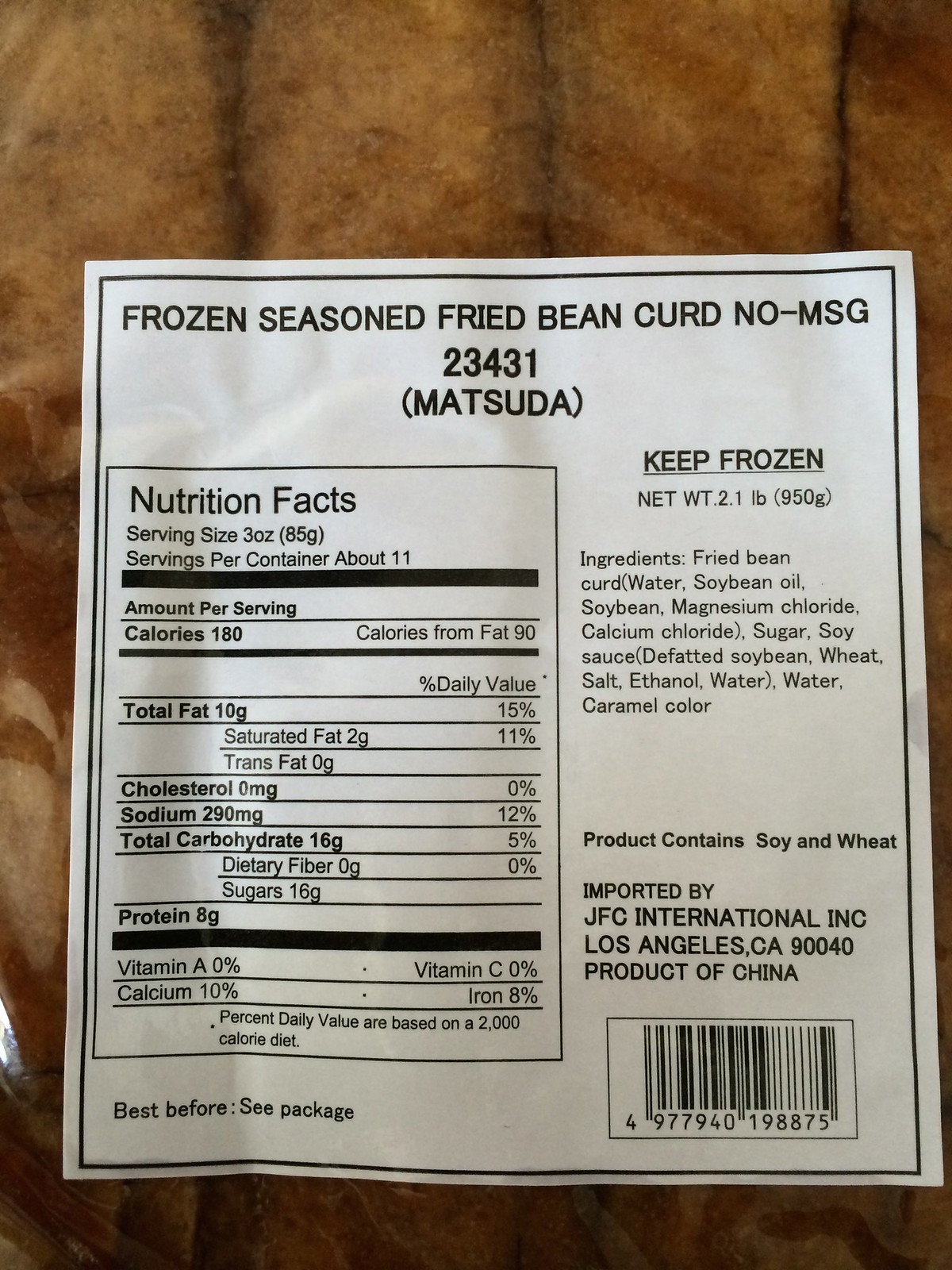This is a detailed close-up color photograph of a food label, which appears against a padded, horizontally-lined brown background with shadows to the left and bottom. The label is primarily white with black text and has a thin black border. The top of the label reads, "Frozen Seed, Seasoned Fried Bean Curd, No MSG, 23431 Matsuma," and to the right of this text, it says, "Keep Frozen." Directly below is the net weight information. The bottom right corner features a barcode. Below this, there's a comprehensive list of ingredients including: fried bean curd, water, soybean oil, soybean magnesium chloride, calcium chloride, sugar, soy sauce (defatted soybean, wheat, salt, ethanol, water), and caramel color. To the left, encased in another narrow box, are the nutritional facts, which detail serving size, servings per container, calories, total fat, cholesterol, sodium, total carbohydrates, protein, along with amounts of vitamin A and calcium. At the very bottom left corner, the label mentions, "Best Before: C Package." Additionally, it notes the product was imported by JFC International Inc., Los Angeles, CA 90040, and is a product of China.